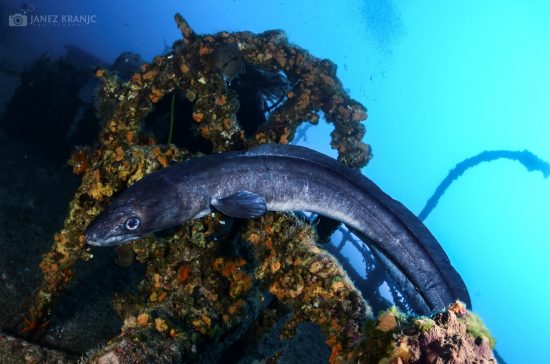This underwater photograph captures a long, eel-like fish swimming gracefully amidst the wreckage of a sunken ship. The fish, approximately three to three and a half feet in length, features a dark gray top, medium gray sides, and a white underbelly, with a large eye and elongated body highlighted by a continuous dorsal fin running along its back. Its twisted form extends from the upper left towards the bottom right of the frame. Behind the fish, the remains of a ship are visible, including a wooden steering wheel encrusted with barnacles, moss, and algae—a testament to its long submersion. The background is filled with a vibrant underwater landscape, with bright blue water illuminating the scene, contrasting with the darker hues on the left. In the top left corner, a watermark bearing the text "Janice Cran JC" is present.